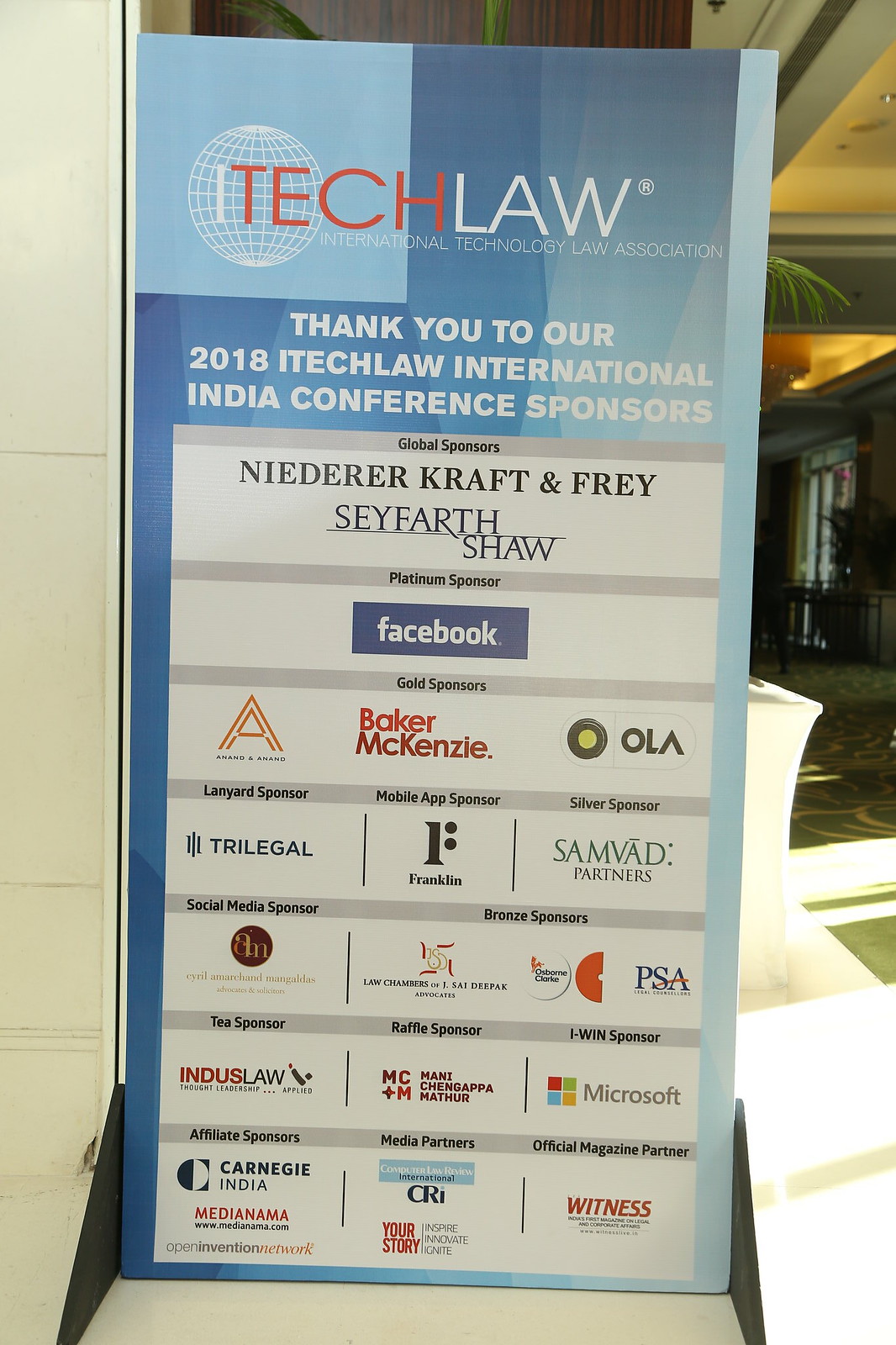The image depicts a tall, slender, vertically-oriented poster prominently placed at the center. The poster is primarily light blue with a blue gradient design and features the heading "Tech Law," with "tech" in red and "law" in white. Below this, a bold white text reads, "Thank you to our 2018 iTech Law International India Conference sponsors," with an array of sponsor logos listed underneath against a white background. Notable sponsors include Facebook, Tyler McKenzie, OLA, and PSA, among others. To the left of the poster is a smooth, off-white tiled wall, while to the right, part of a hallway with a green and yellow patterned carpet and a green ceiling is visible. The top right corner of the image shows the tip of a plant leaf peeking out from behind the poster, indicating the conference setting.